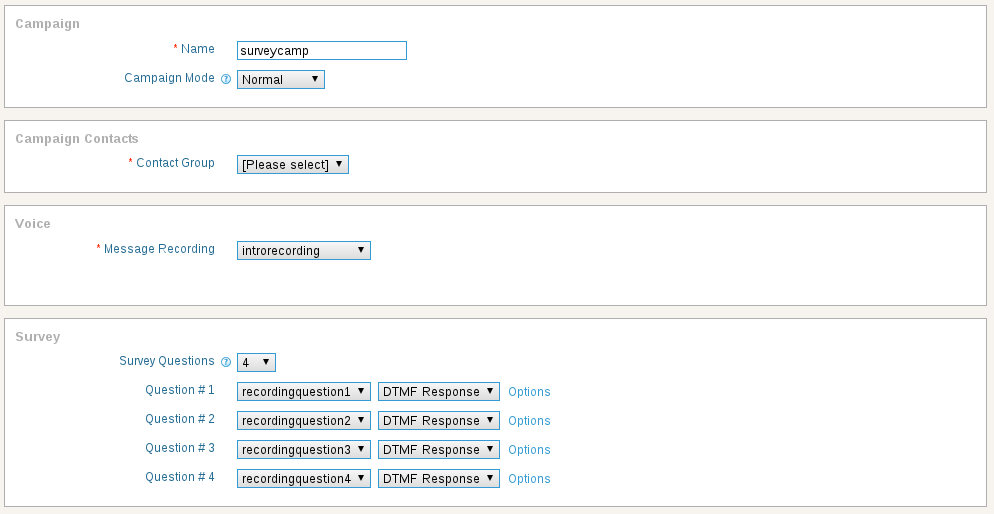The image depicts a user interface for setting up a campaign, possibly for advertising or survey purposes. The layout is primarily on the left side of the screen, while the right side remains empty, extending significantly to the right.

**Top Section: Campaign Setup**
- **Campaign Details**: 
  - A horizontal, white rectangular box labeled "Campaign" in gray.
  - Below it, a blue-labeled field titled "Name," with the input field outlined in blue displaying "Survey Camp."
- **Campaign Mode**: 
  - A label "Campaign Mode" is followed by a dropdown menu displaying "Normal."

**Middle Section: Campaign Contacts**
- **Contacts and Groups**:
  - A white box labeled "Campaign Contacts."
  - Below it, a field titled "Campaign Group" with a dropdown menu prompting "Please select."

**Voice Section**
- **Message Recording**:
  - A white box labeled "Voice."
  - Inside, a label "Message Recording" is followed by a dropdown menu displaying "Intro Recording."

**Survey Section**
- **Survey Setup**:
  - A white box labeled "Survey."
  - Inside, a label "Survey Questions" with a dropdown menu indicating "4."

For each question within the survey:
- **Question One**:
  - "Recording Question 1" with an adjacent dropdown menu.
  - "DTMF Response" with a neighboring dropdown menu.
  - An "Options" label in blue next to it.
- **Question Two**:
  - "Recording Question 2" with an adjacent dropdown menu.
  - "DTMF Response" with neighboring dropdown menus.
  - Blue "Options" label.
- **Question Three**:
  - "Recording Question 3" with an adjacent dropdown menu.
  - "DTMF Response" with neighboring dropdown menus.
  - Blue "Options" label.

This detailed description maps out the structure and content of the campaign setup interface, highlighting the areas for input and selection within the different sections of the form.